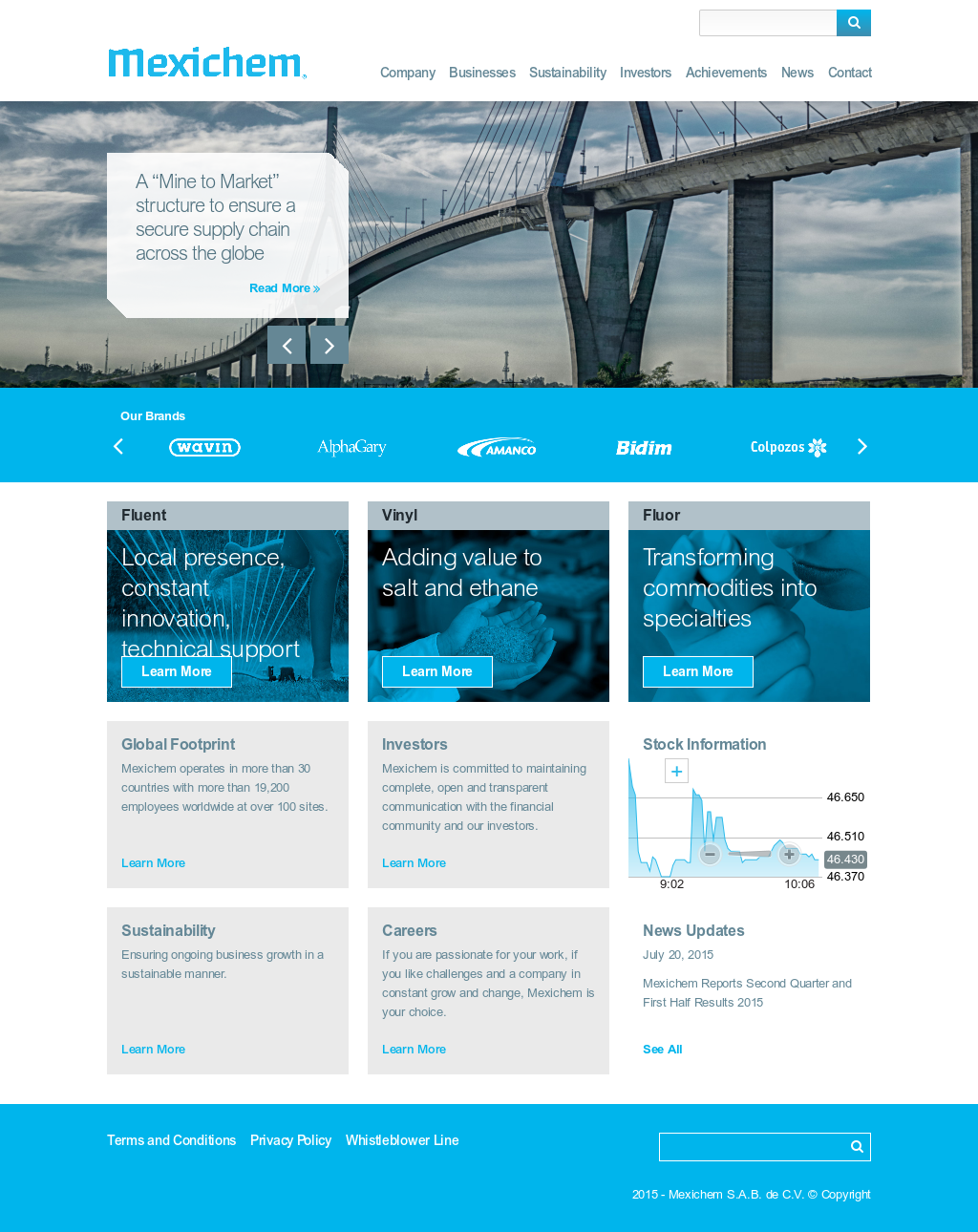The website features a predominantly white background accentuated with a very light blue color scheme. At the top left corner, the brand name "Mexichem" is prominently displayed. Adjacent to this, a horizontal navigation menu offers various sections, labeled as Company, Business, Sustainability, Investors, Achievements, News, and Contact.

Below the menu, there's a large image showcasing an extensive traffic bridge, accompanied by the caption "Mine to market structure to ensure a secure supply chain across the globe."

Below this image, four succinctly titled boxes are aligned horizontally:
1. **Local Presence, Constant Innovation, Technical Support** - Labeled "Fluent"
2. **Vinyl** - Featuring the tagline "Adding value to salt and ethane"
3. **Fluor** - Highlighted with the description "Transforming commodities into specialties"

Further down, there are two rows, each consisting of three smaller squares filled with additional information. These boxes cover topics such as Sustainability, Careers, News Updates, Stock Information, Investors, and the company's Global Footprint. 

At the very bottom of the page, a blue bar spans the width of the site, possibly housing additional navigational links or contact information.